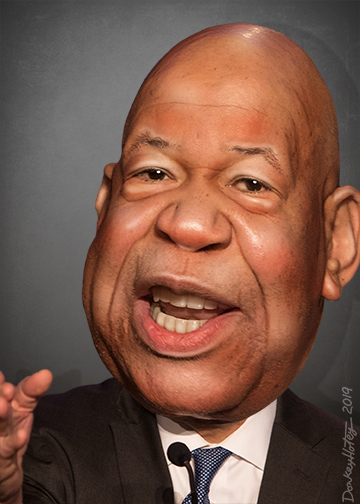This image is a vertically aligned rectangular caricature of a middle-aged African-American man with distinctive features and a nuanced background. The man is bald and has a somewhat chubby face, which broadens towards his cheeks and sides, emphasizing his expressive and smiling demeanor as he speaks, revealing both his top and bottom white teeth. His eyes are a deep brown, and his expression suggests he might be addressing an audience. 

He is dressed in a sharp black suit jacket paired with a white collared button-down shirt and a patterned blue tie adorned with white dots. A small black microphone is clipped to his tie, positioned near the center of his chest. The caricature's head is disproportionately large, roughly five times bigger than typical for the size of his suit and shoulders, drawing attention to his amplified facial features including his large ears.

In the lower left corner of the image, a small hand is visible, likely making a gesture. The background features a gradient that transitions from light gray to black, adding a subtle contrast to the composition. Along the right side of the image, vertically printed in gray, reads "Donkey Hoats 2019," which is presumably the artist's signature.